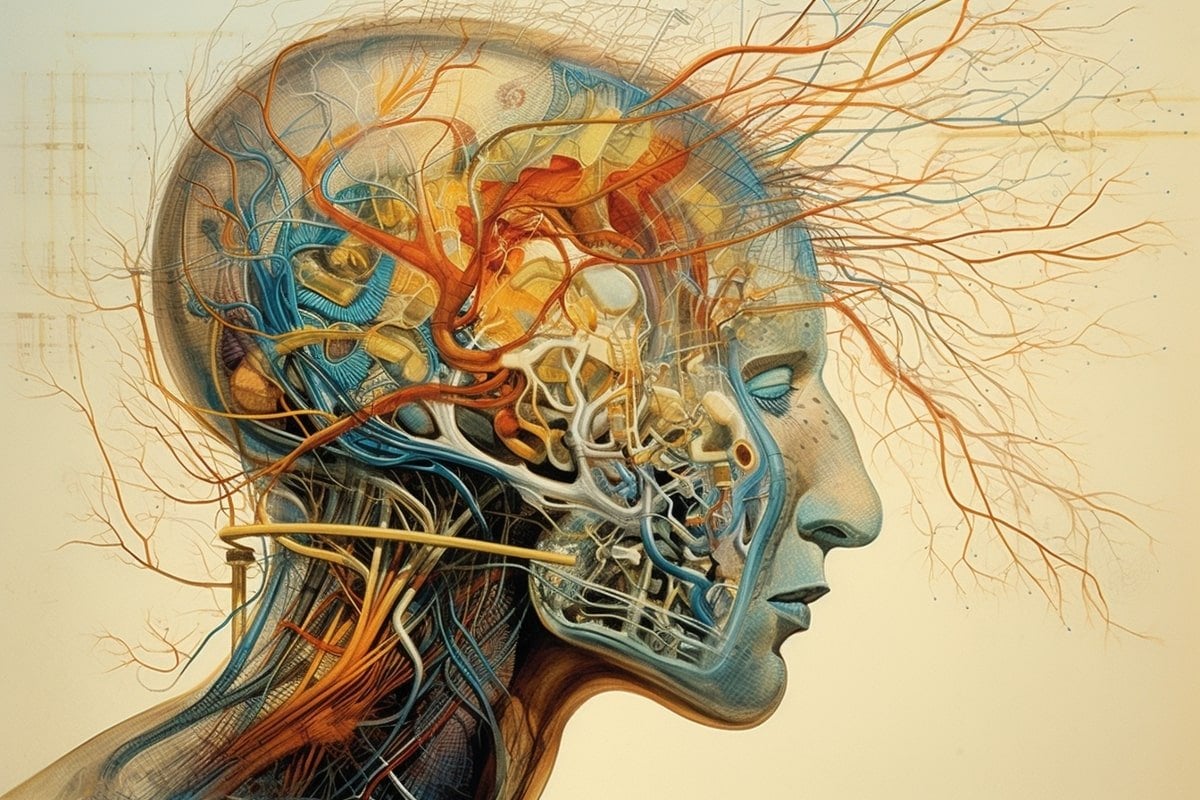This detailed illustration, rendered on a rectangular, light tan brown background shifting to a grayish tone with crisscross patterns towards the upper left corner, depicts the side view of a human head and neck. The head, devoid of hair and featuring a nose with a slight bump and closed eyes, shows elements of both anatomical and abstract art. The profile of the face is shaded in blue and sprinkled with freckles. Inside the transparent side of the head, an intricate, imaginative network of veins, resembling tree branches in hues of blue, red, orange, yellow, and white, extends from the skull and intertwines with the neck. These colored veins intertwine like tendons or the nervous system, expanding up and outwards, with branches fanning out along the forehead. The lower jaw appears to be held in place by wire-like structures extending up into an unconventional depiction of the brain, represented by a complex tangle of colorful cords. The entire image, potentially created with colored pencils, gives an impression of a vibrant and dynamic inner life, merging biological and surreal elements.